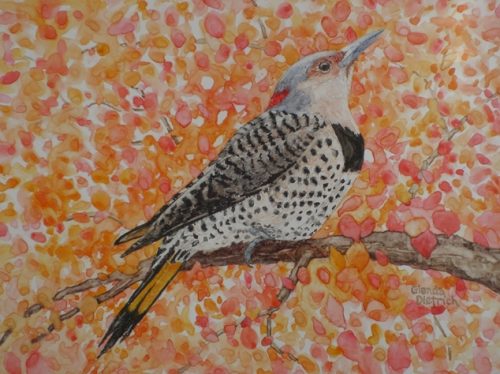This image is a detailed painting of a bird perched on a branch, set against a vibrant background of watercolor dots in shades of peach, orange, light pink, and dark pink, filling the entire canvas. The branch, painted in brown, stretches horizontally across the image, with the bird perched prominently upon it. The bird itself is realistic and intricately detailed, featuring a mostly white belly adorned with black speckles, a small portion of black on its chest, and gray and black striped wings. Its head is primarily white with some gray on the back and a striking strip of bright red. The bird's beak is pale gray, and its eyes are encircled with red. Notably, the bird is looking up to the upper right-hand corner, with its tail pointed downwards and ending in yellow feathers tipped in black. The background's watercolor dots create an impressionistic feel, reminiscent of autumn leaves either falling or about to fall. Finally, there’s a signature watermark in the bottom right-hand corner, adding an element of authenticity to the artwork.